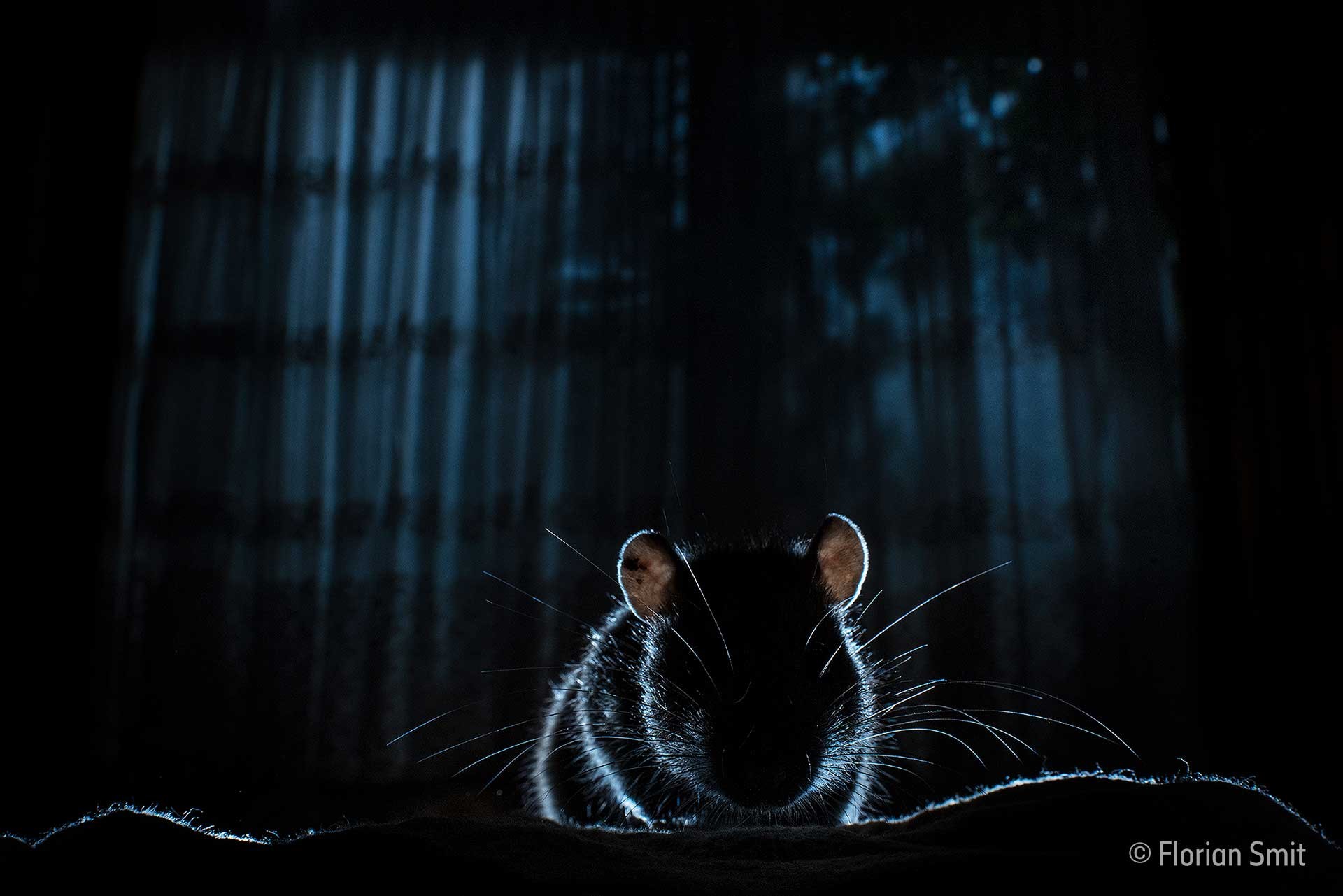In this atmospheric photograph, a dark mouse or rat stands on some kind of sheet or blanket against a deeply shadowed background that transitions from blackish-blue at the top to nearly pitch black at the bottom. The mouse is almost camouflaged with the darkness, with only the delicate outlines of its ears, whiskers, and body faintly illuminated by an unseen light source, casting a bluish glow. Its face is obscured, leaving only its contours visible. Behind the mouse, the setting appears to be an indoor room with a window featuring panes and a semi-transparent curtain. Outside the window, silhouetted tree leaves are faintly visible against the dark night sky. The scene is given a mystic, nocturnal ambiance, further credited at the bottom right with "C. Florian Smit."